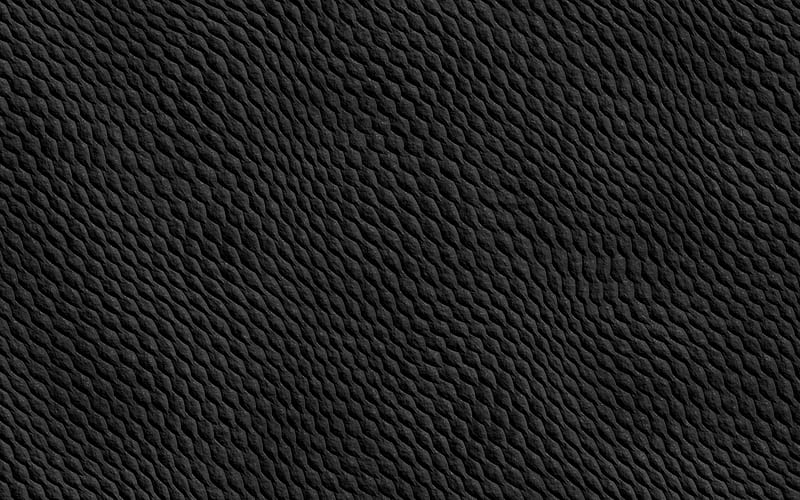The image features a close-up of a textured, dark gray material that covers the entire frame. The material appears reminiscent of animal skin, such as a crocodile or snake, due to its rough and pattern-like surface but is more uniform, lacking distinct markings. The texture forms an intricate, marquise-cut pattern that looks somewhat like interlocking diamond shapes. These shapes create a series of rivulets running diagonally from the top left corner to the bottom right. These rivulets do not run parallel; instead, they interlock in a manner where one line's curve fits into the adjacent one, creating areas that appear alternately compressed and expanded. The overall effect resembles a fabric-like material, possibly a rug, towel, tablecloth, or wall covering, in a shade that ranges from dark gray to nearly black.